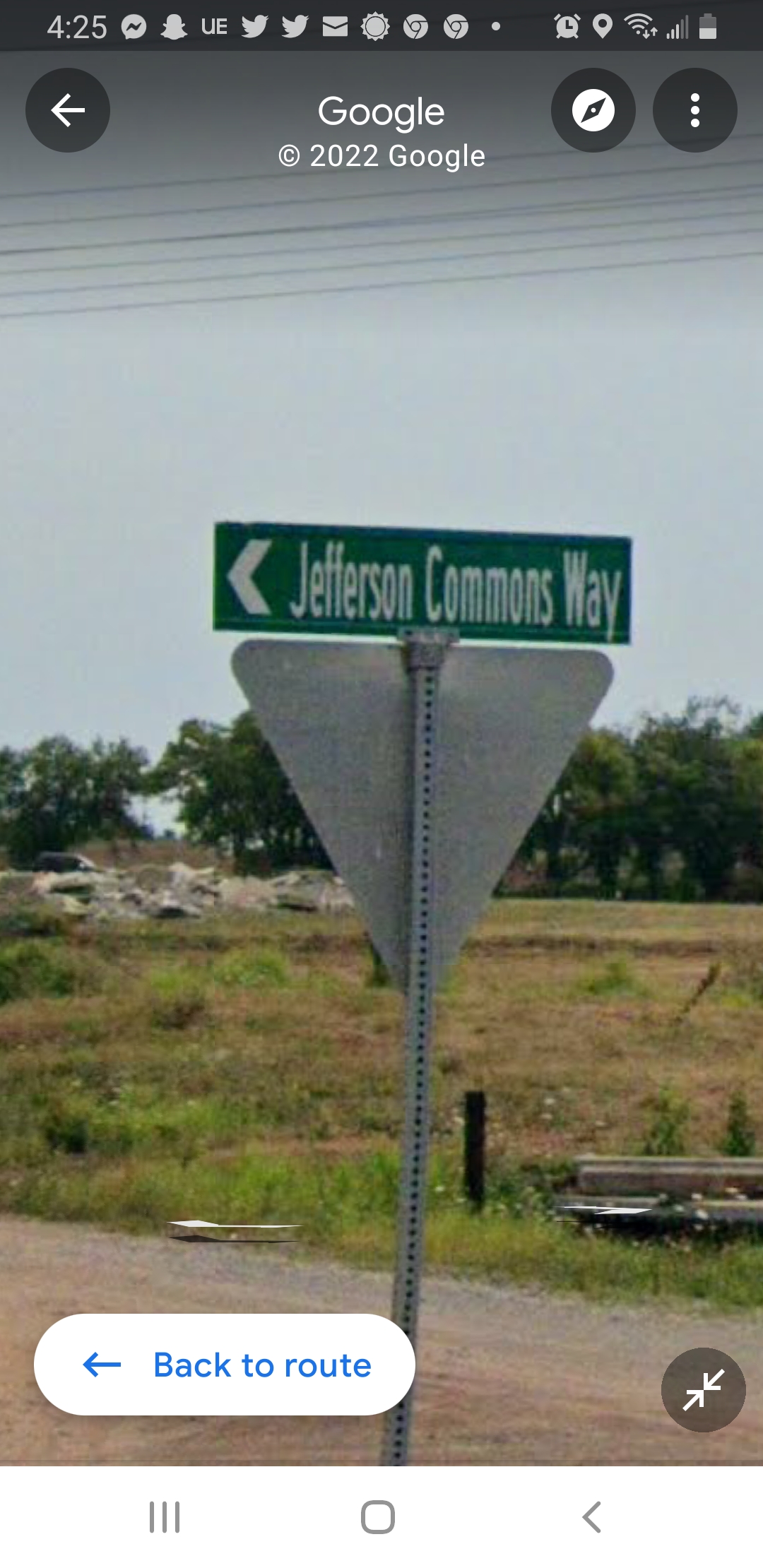The image depicts a rural scene captured in Google Street View, as indicated by the "Google copyright 2022 Google" text prominently displayed at the top of the screen. The image has various app icons along the top, such as Messenger, TikTok, and Twitter, making it apparent that the screenshot is taken through a phone in portrait mode. The main focus of the photo is a rural dirt road with bits of gravel, surrounded by scrubland and a distant bank of trees under a gray sky. Centrally positioned is a metal pole holding a green, rectangular street sign. The sign, with white letters, reads "Jefferson Commons Way" and includes a left-pointing arrow. Just below it is the back side of a yield sign, characterized by an upside-down triangular shape and a silver exterior. Additionally, at the bottom left of the screen interface, there is a white and blue "Back to Route" button, alongside other on-screen navigation icons. The combination of signs and surrounding environment seamlessly conveys the tranquil and undeveloped nature of this rural area.